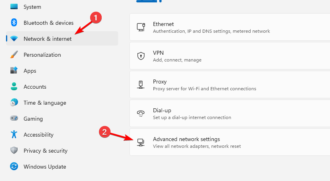Caption: 

This image showcases the settings interface of a device, possibly a phone or a computer. The screen is divided into two vertical sections, with the left-hand sidebar listing various categories such as System, Bluetooth and Devices, Network and Internet, Personalization, Apps, and several others that include Accounts, Time and Language, Gaming, Accessibility, Privacy and Security, and Windows Update. The 'Network and Internet' category is highlighted, indicated by a red arrow and labeled with a red circle containing the number '1'. This highlights the selected section in the left sidebar. On the right-hand side, detailed options corresponding to the 'Network and Internet' category are displayed. These options include Ethernet, VPN, Proxy, Dial-Up, and Advanced Network Settings. Another red arrow, labeled with a red circle containing the number '2', points to the 'Advanced Network Settings' option, which allows users to view and manage all network settings.